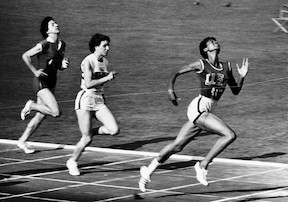This black-and-white photograph captures a dramatic moment in a track race, possibly a collegiate event. It features three female runners, all with dark hair, sprinting toward the finish line. The leading runner, dressed in a dark shirt, white shorts, and white sneakers, is about to break the finish line's string, which stretches tautly across her chest. Close behind her, the second runner sports a white shirt, white shorts, and white sneakers, while the third, trailing behind, wears a dark outfit—both shirt and shorts—with white sneakers. The race is taking place on a paved track encircling a grass infield, which occupies much of the photograph's upper half. A folding chair is visible off to the upper right, adding a touch of casual observation to this otherwise intense athletic moment.